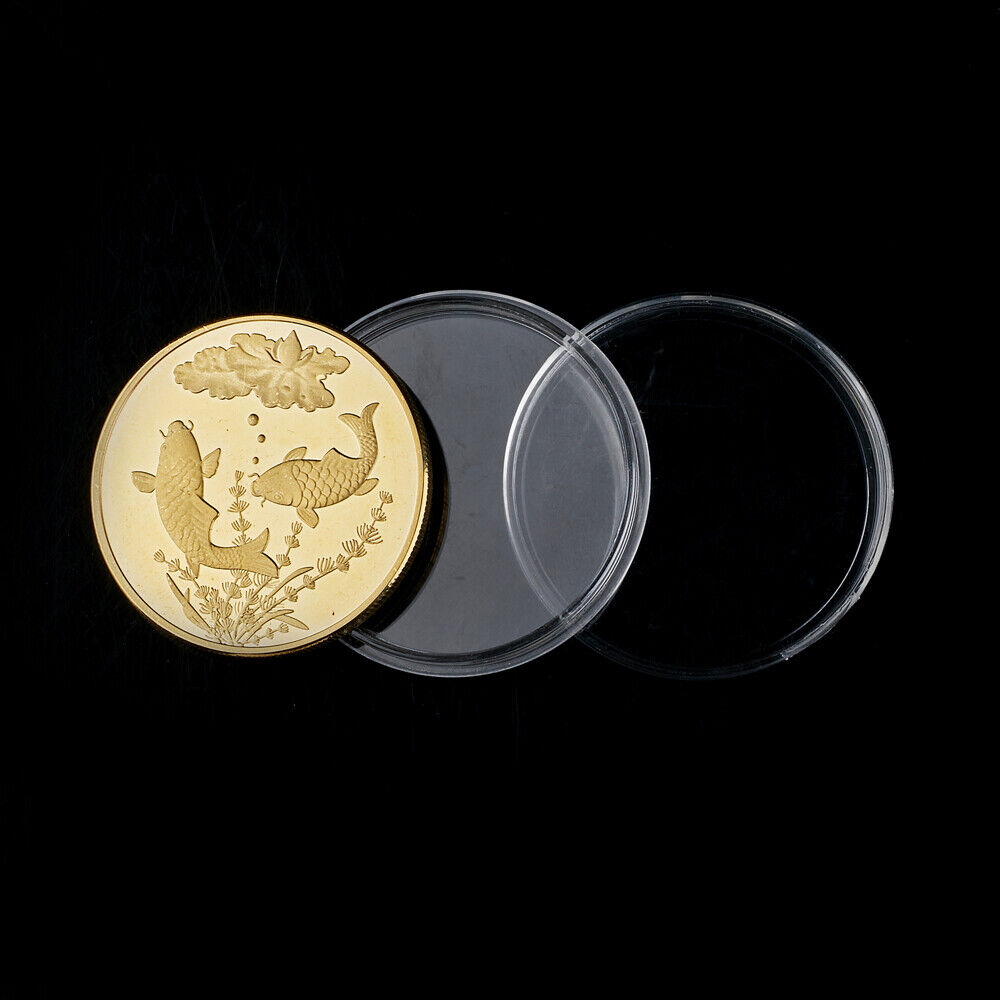In the photograph, set against a completely black background, there is a clear circular plastic container prominently displayed. The lid of the container is situated to the side, leaning against the bottom part of the dish. Adjacent to the container, on the left side, rests a bright shiny gold coin. This coin features intricately raised designs depicting two koi fish: one positioned on the left and curved towards the right, and the other on the right curving towards the left. Above the koi fish is a detailed lotus flower, while below them, there are seaweed-like plants sprouting upwards. The right fish also has three small bubbles rising from its mouth. The coin itself has a raised, ridged edge. The clear container and its lid appear to be fitted perfectly to securely encase this ornamental coin.